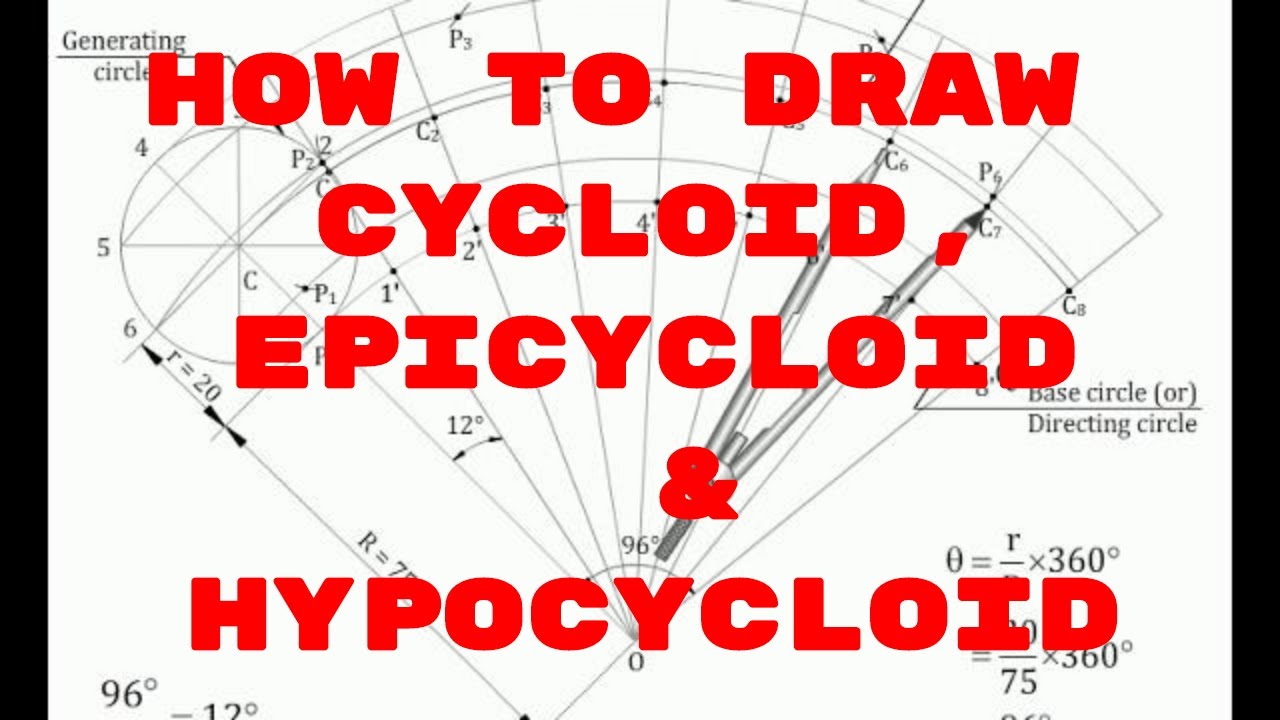The image features a pristine white background adorned with a meticulously detailed protractor drawing, which illustrates the creation of various mathematical curves. Central to the composition is a prominently displayed title in bold red typography that reads, "How to Draw Cycloid, Epicycloid, & Hypocycloid," where the ampersand symbol is predominantly filled in due to the font style. The diagram meticulously delineates the geometric configurations involved, including the generation of circles—specifically, the base circle and the directing circle—as well as comprehensive math computations that accompany these constructions. Several degree markings are visible, enhancing the precision and instructional quality of the illustration. Additionally, a gray, pencil-drawn protractor, designed to mimic a silver protractor, is depicted within the diagram, emphasizing the practical tools needed to recreate the curves. This detailed visualization serves both as an educational tool and a graphical representation of advanced geometric concepts.